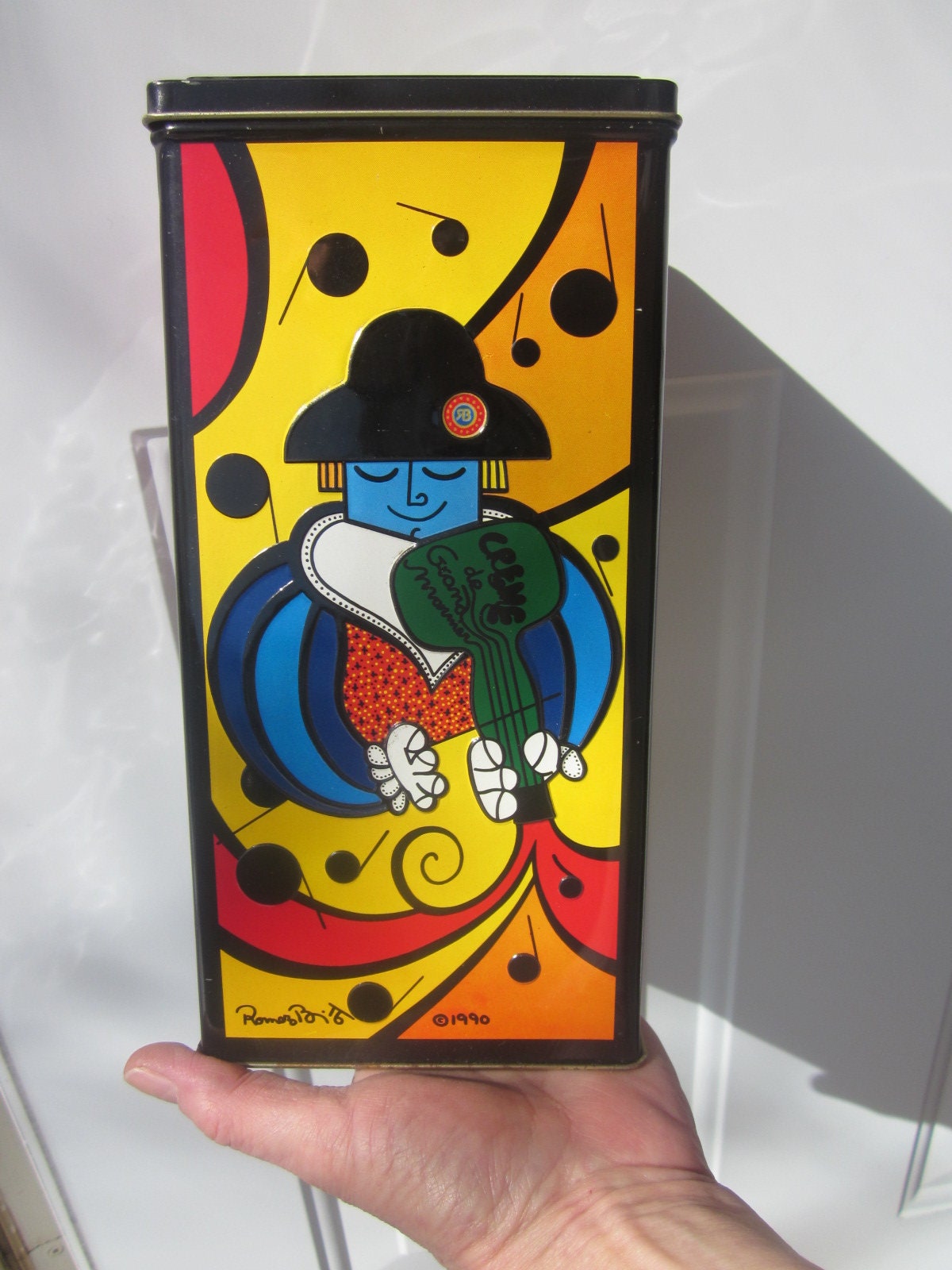A detailed and combined caption for the image:

In this photograph, a left hand is extended, holding a tall, rectangular metallic tin container with a black lid featuring a silver outline. The front of the container showcases vibrant, pop urban artwork, depicting a blue-skinned cartoon character resembling a musician. The character wears a black hat and a two-tone blue outfit with a white bib. In his right hand, he carries a green guitar. Surrounding the character are swirling patterns in shades of orange, red, yellow, and mustard, creating a dynamic background. Scattered around the character are black musical notes. The box, possibly identified as “crème de grande,” could be a European liqueur container, contributing to its artistic and cultural aesthetic.